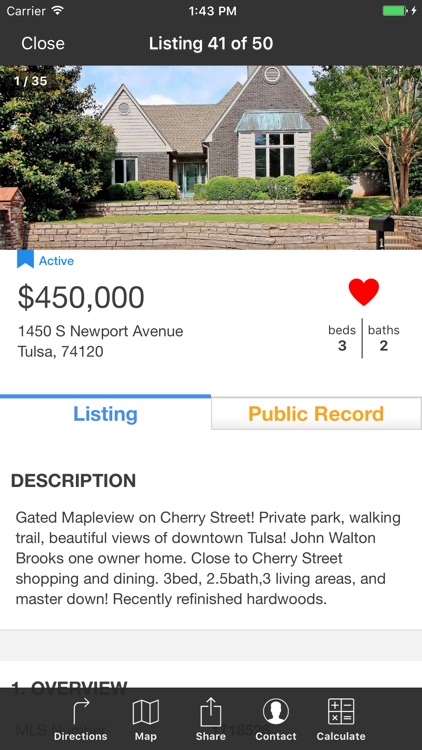**Detailed House Listing Screenshot Description**

At the top of this mobile screenshot, a black border typical of mobile devices displays various icons and text. On the top left, the word "carrier" is visible next to a Wi-Fi symbol. Centered at the top, the time is shown in white as 1:43 PM. On the far right, a green battery icon, almost full, is accompanied by a white lightning bolt symbol.

Below the black border, the image states "Listing 41 of 50" at the center, with "closed" located on the left under the carrier information. Dominating the screen right below this text is a picture of a house featuring two pointed gray roofs, white window shutters, and surrounding trees. A brick border frames the lawn of the house.

In the subsequent section underneath the house picture, a blue bookmark icon on the top left indicates "active" status. Adjacent to this, the price is listed prominently against a white background as $450,000. Directly below, the address reads "1450 South Newport Avenue, Tulsa, 74120". On the right side of this section is a red heart symbol with the specifications "beds: 3" and "baths: 2" listed below it, separated by a vertical line.

Toward the bottom, two tabs offer additional information. The selected "listing" tab is highlighted in blue with a line above it, while the "public record" tab is marked in yellow. In the "listing" tab, bold black font denotes "Description", followed by a smaller paragraph detailing the property's features: "Gated Maple View on Cherry Street, private park, walking trail, beautiful views of downtown Tulsa, John Walton Brooks, one owner home, close to Cherry Street shopping and dining, three beds, 2.5 baths, three living areas and master down, recently finished hardwood."

A light gray separator provides some spacing before the next white box section labeled "Overview". It lists the MLS number on the right, partially obscured by a semi-transparent black navigation menu, showing "1718526". This navigation menu includes directional icons and options for "Direction," "Map," "Share," "Contact," and "Calculate," each having their corresponding icons.

A comprehensive depiction of the house listing, all specifics, and navigation options are clearly presented within this mobile screenshot.